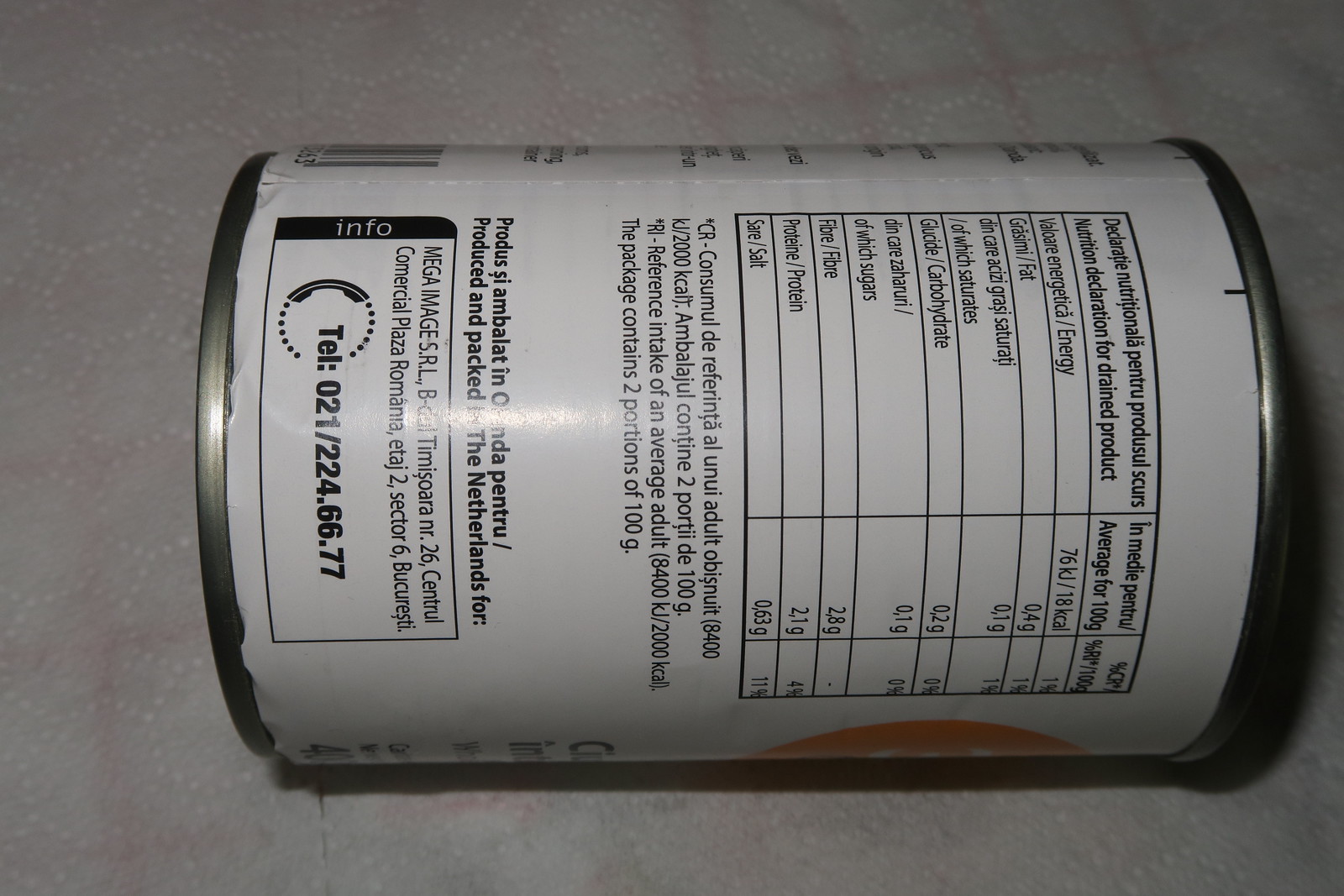A detailed side view of a can's nutritional panel is captured in this horizontal photograph. The can appears sideways, displaying the back label prominently. The nutritional information, along with other textual details, is printed in a foreign language, and the panel is positioned near the top of the can. Centrally located below this section is an asterisk accompanied by additional information. At the bottom of the label, a telephone number is provided for contact. The label itself is white and features a distinctive orange semicircle located towards what would be the bottom right corner of the label from this perspective. The can rests on a white paper towel, revealing the towel's textured, quilted design.